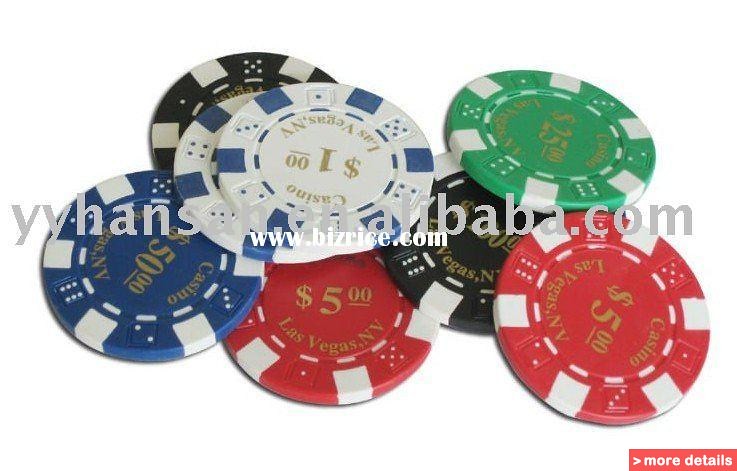This is a highly detailed color photograph of a pile of poker chips, typically used in casinos, set against a completely white background. The chips are scattered in the pile, with a black chip positioned at the very bottom, followed by another black chip and a red chip. Higher in the pile, a blue chip, another black chip, and two white chips can be seen. A green chip and another red chip sit prominently towards the top. Each chip has a designated value: the red chips represent $5, the blue chip is $50, the white chips are $1, the green chip is $25, and the black chips are $100. Superimposed in the foreground is the website URL www.bizrice.com, while a small section at the bottom right showcases a red banner with the text "More Details" in white, indicating that additional information can be accessed. This composition appears to be primarily designed for advertising purposes, prominently featuring the website and the detailed, colorful assortment of poker chips.